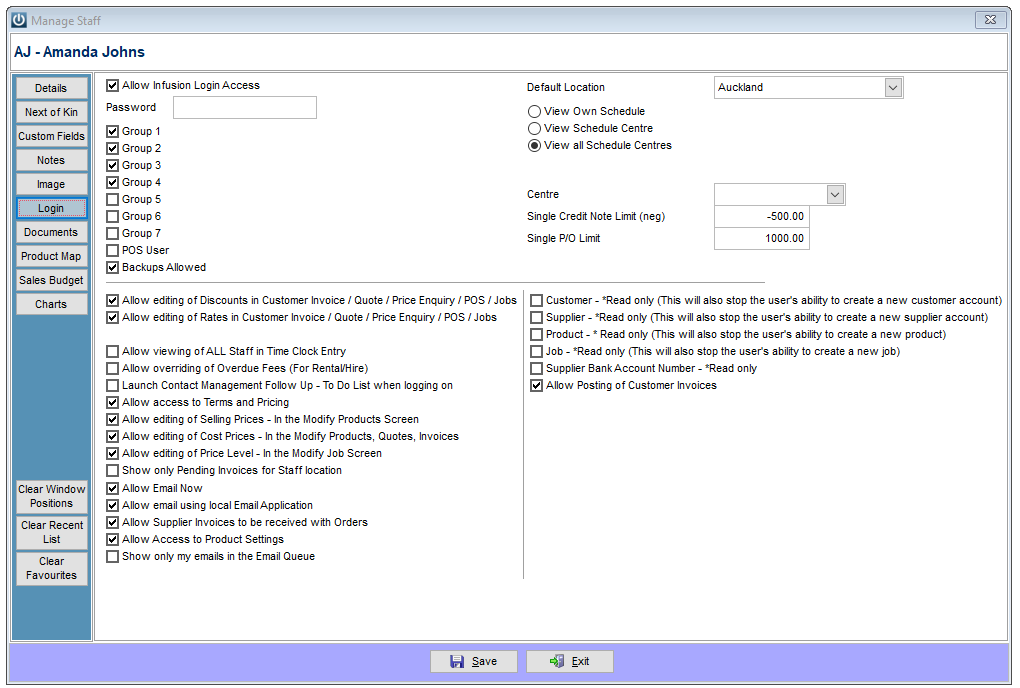**Caption:**

This image is a screenshot likely captured from a desktop or laptop screen showcasing a staff management software interface. 

At the top, there is a silver taskbar. On the top left of this taskbar, a power icon is visible, and to its right, the text "Manage Staff" is displayed. Just below, it reads "AJ-Amanda Johns".

On the left side of the window, a light blue column houses several gray tabs with black text. These tabs are labeled as follows: Details, Next of Kin, Custom Fields, Notes, Image, Login (highlighted in light blue and written in blue text), Documents, Product Map, Sales, Budget, and Charts. Further down, with a small gap separating them, are options labeled Clear Window Positions, Clear Recent Lists, and Clear Favorites.

The main body of the window features a predominantly white background with several black text entries and checkboxes. At the top of this section, there is a checkbox labeled "Allow Infusion Login Access." Directly beneath this is the text "Default Location: Auckland" and below that, a password box.

Further below, several group options are listed with checkboxes: Groups 1 through 4 are checked, while Groups 5 through 7 and POS User are unchecked. There is also an option labeled "Backups Allowed" which is ticked.

On the right side, underneath "Default Location," additional options appear. These include:
- "View Own Schedule" (unchecked),
- "View Schedule Center" (unchecked),
- "View All Schedule Centers" (checked).

Below this section, a drop-down menu under "Center" appears. Additional selections include:
- "Single Credit Note" indicating a negative value of -500,
- "Single P-O limit" indicating a value of 1,000.

A list of permissions follows, including checkboxes that indicate what staff can do:
- "Allow Editing of Discounts and Customer Invoice, Quote Price Inquiry, POS, and Jobs" (checked),
- "Allow Editing of Rates and Customer Invoice, Quote Price Inquiry, POS, and Jobs" (checked),
- Several unchecked items such as "Allow Viewing of All Staff in Time Clock Entry," "Allow Overriding of Overdue Fees (for Rental/Hire)," "Launch Contact Management," and "Follow Up To-Do List when Logging On."

The interface appears to be a comprehensive and detailed staff management software platform. At the bottom of the window, in a light purple lilac background, there are two distinct buttons labeled "Save" and "Exit."